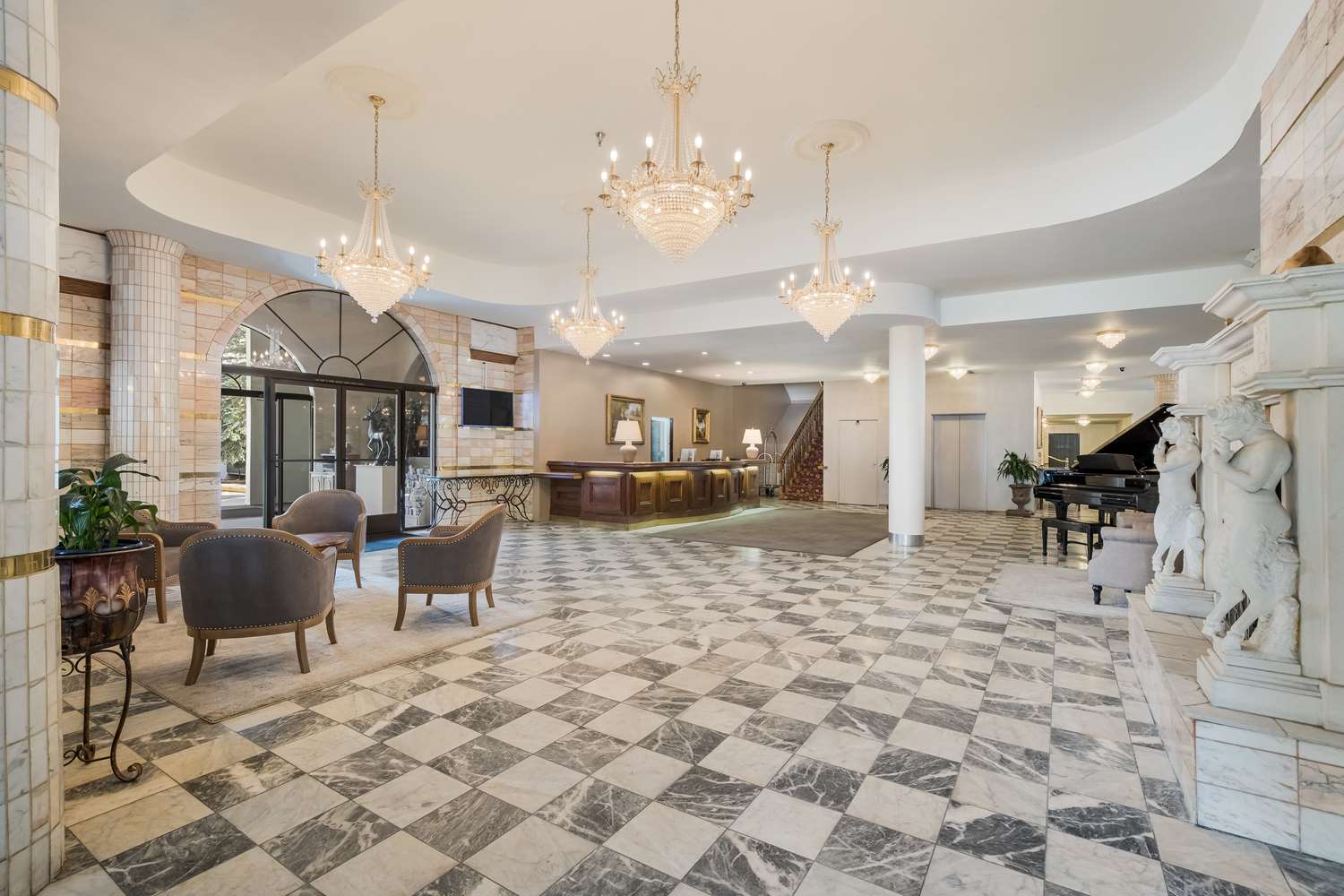This photograph captures the grand lobby of what appears to be a luxurious mansion or high-end hotel. The area features elegant gray and white checkered marble or granite flooring, extending throughout the space. Dominating the right side is a large fireplace, flanked by intricate sculptures resembling ancient Greek figures with the lower halves of horses and upper bodies of humans. Adjacent to the fireplace stands a black grand piano, accentuating the opulent setting.

The back wall showcases two elevators framed by planters, with a grey area rug leading up to them, and a staircase that ascends to an upper level. To the left of the elevators is a stately reception desk under a set of smaller recessed lights in the white ceiling. The ceiling also houses four stunning white or gold chandeliers, casting a warm glow over the entire room.

On the left side, near the large glass arched doorway that offers a glimpse outside, comfortable plush gray armchairs are arranged in a cozy seating area with a cream-colored rug underneath. A decorative urn holding vibrant green plants adds a touch of nature to the sophisticated space. 

Overall, the room exudes a sense of refined elegance and grandeur, combining luxurious materials and detailed decor to create a stunningly impressive environment.